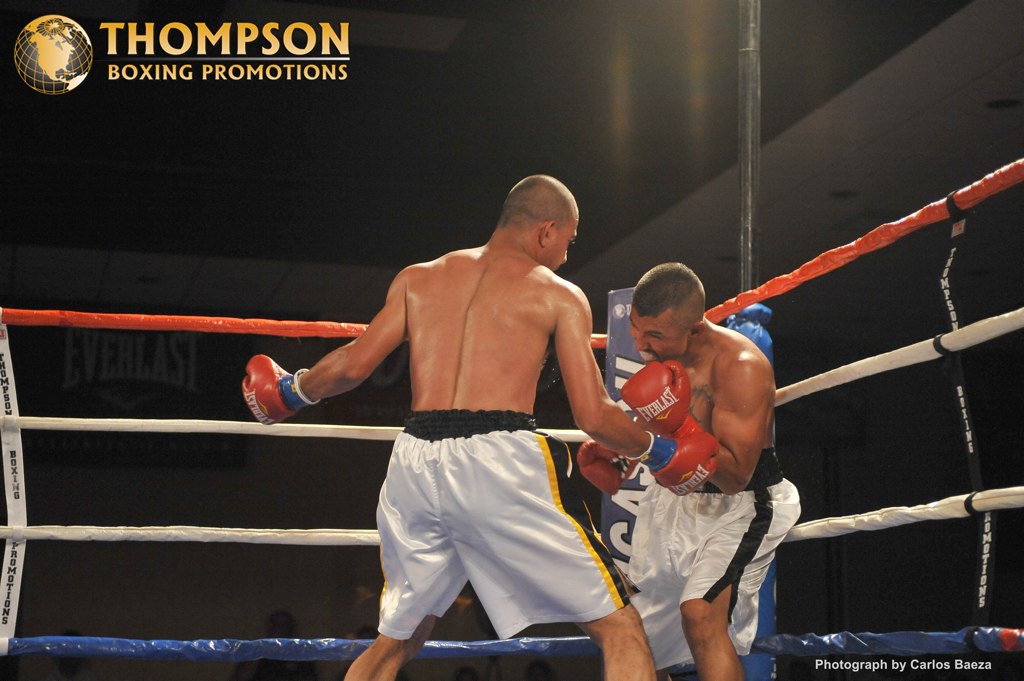This detailed image captures an intense boxing match under the auspices of Thompson Boxing Promotions. The photograph, taken by Carlos Beza, features two dark-skinned boxers centrally positioned in a brightly lit boxing ring, which contrasts sharply against the dark, possibly nighttime, background. The boxer on the left, seen from behind, sports black and white shorts with gold trim, while the opponent on the right, facing the camera, wears black and white shorts. Both athletes don red Everlast boxing gloves, with the boxer on the left also wearing blue wrist tape.

The ring's ropes are vividly colored in red, white, and blue, extending diagonally from a corner just right of the center to the image's edge, marking the ring's boundary amid a backdrop that includes a tiled ceiling and a wall. Above the fighters, a globe and the text "Thompson Boxing Promotions," both in gold, occupy the top left of the black background, prominently displaying the event's branding. The entire scene is grounded on a platform enclosed by the ropes, creating a dynamic and taut atmosphere of competitive sportsmanship.